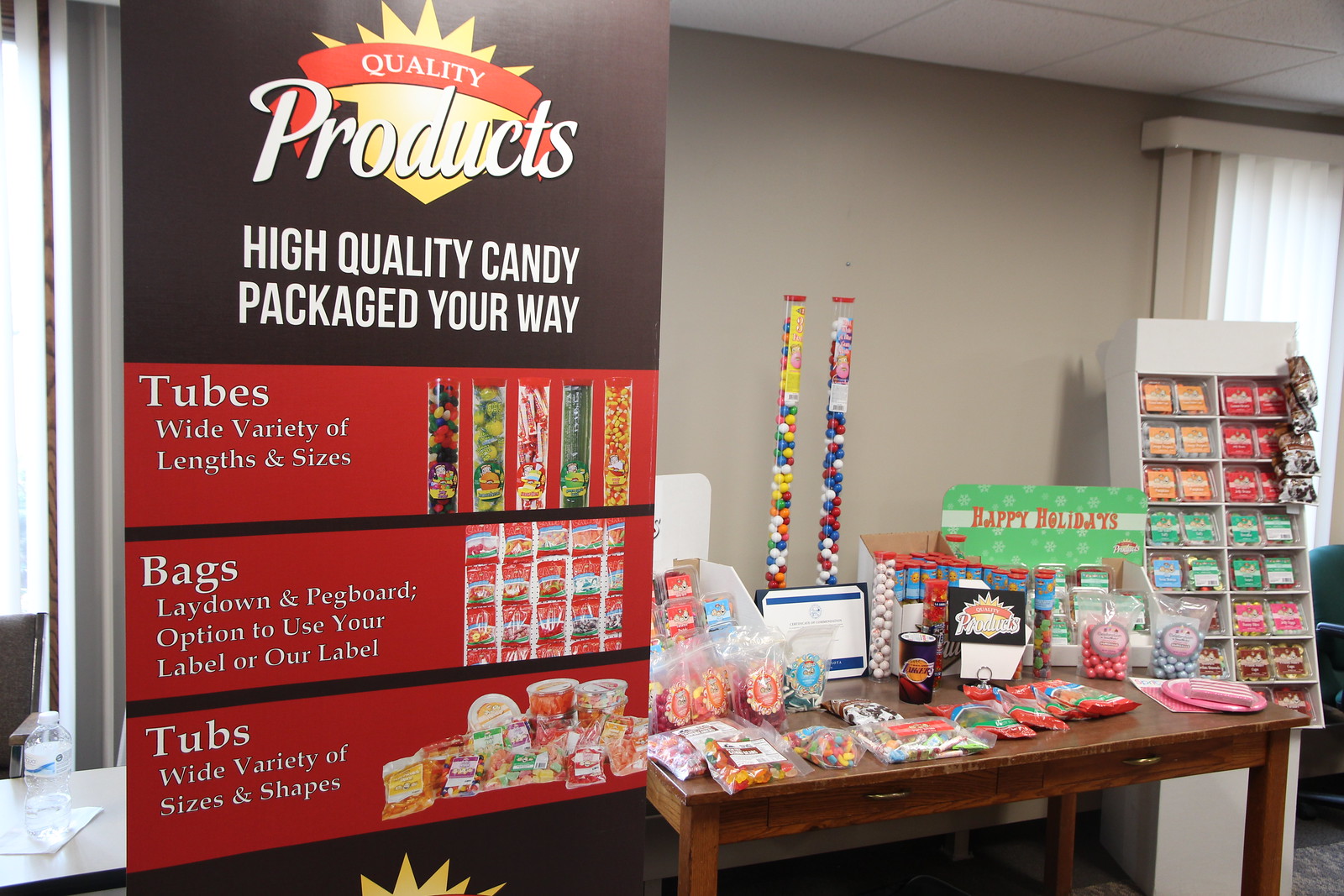The photograph depicts a detailed display setup at a candy store, centered around a brown wooden table with two drawers. The table is arranged with an assortment of snacks, including various bags, tubes, and tubs of candy, chips, and other sweets. To the right of the table stands a white display shelf showcasing additional bags, boxes, and containers of candy. Prominently featured on the table is a sign with red lettering on a green background that reads "Happy Holidays." At the back of the table, two tall containers of gumballs add a festive touch.

On the left side of the table, there is a large, vertically oriented sign designed to look like a crown. This sign features multiple sections: the top part is black, and the main information displayed is in red on a yellow background with a crown-like design. The sign reads "Quality Products" in large white letters, followed by the tagline "High Quality Candy Packaged Your Way." Below this, the sign details various packaging options – "Tubes," illustrated with images of various lengths and sizes; "Bags," with images showing both lay-down and pegboard options; and "Tubs," highlighting a wide variety of sizes and shapes. The setting is further described with a white wall in the background, a window adorned with white curtains, and a gray floor below. This immersive display effectively promotes the range of candy products available.